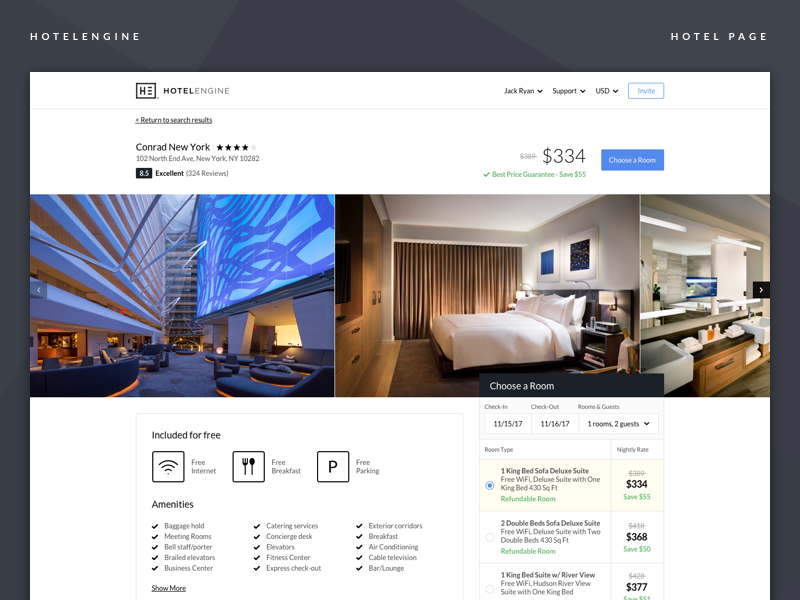The image showcases a website interface with a dark gray, almost black header. On the left side of the header, the words "HOTEL ENGINE" are prominently displayed in bold, white, capital letters. On the right side of the header, the words "HOTEL PAGE" appear, also in white, capital letters. 

Beneath this header is a main white background that features three distinct images. The first image depicts a waiting area furnished with blue-cushioned couches and blue accents at the top. The second image displays a well-made bed in a bedroom, accompanied by a desk situated next to it. The third image illustrates a set of drawers, suggesting it is part of a bathroom setup.

At the bottom, the text "Conrad, New York" is clearly visible, accompanied by a rating of four stars. The price for a stay is listed as $334.